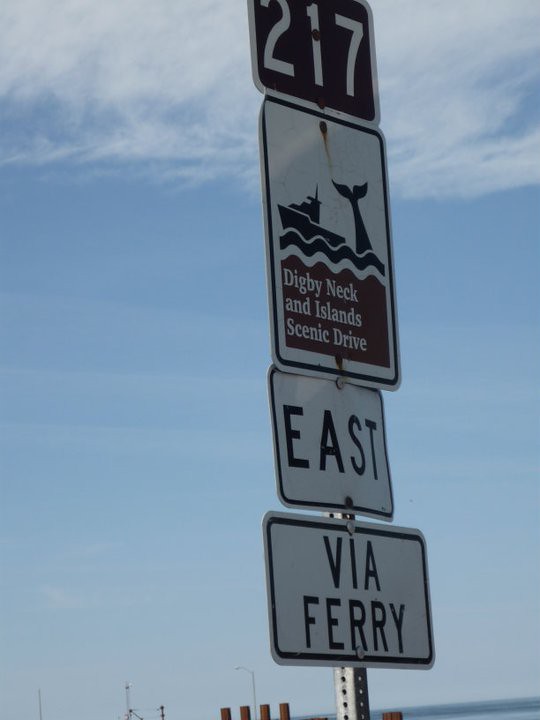This photograph captures four vertically stacked road signs mounted on a perforated silver metal post by an oceanic body of water. At the top, a rectangular black sign with white lettering reads "217," featuring a bolt through the number one. Below it, a sign with a scenic illustration of a boat and a whale's tail in black on a white background reads "Digby Neck and Island Scenic Drive," showing rust from a nail at its top. The third sign is a white square with black capital letters that says "East," and the bottommost sign, slightly wider and rectangular, also in white with black capital letters, reads "Via Ferry." The background showcases a blue sky with wispy cirrus clouds and a slight banding effect. The horizon, slightly lower on the left, reveals smoke stacks, various boat antennas, and a couple of streetlights.